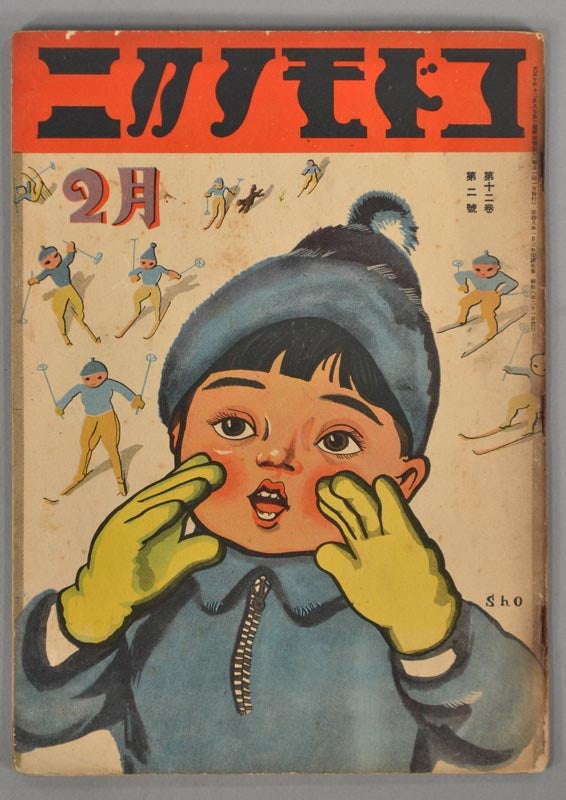The book cover photograph features an old, aged-looking book with a prominent orange banner at the top displaying the title in an unrecognizable language, possibly Japanese or Chinese. The cover itself has a white background adorned with various graphics depicting people skiing down a slope. At the forefront is a detailed drawing of a young Asian girl visible from the chest up. She wears a long-sleeved blue coat or parka with a three-quarter-length zipper that is fully zipped up. Her hands, clad in bright yellow gloves, are raised to her mouth, giving the impression she is shouting. Atop her head sits a blue, fur-like hat with a white puffball, and her black bangs peek out from under the hat. In the background, individuals in yellow pants and blue sweaters are seen skiing, adding to the dynamic, wintry scene.